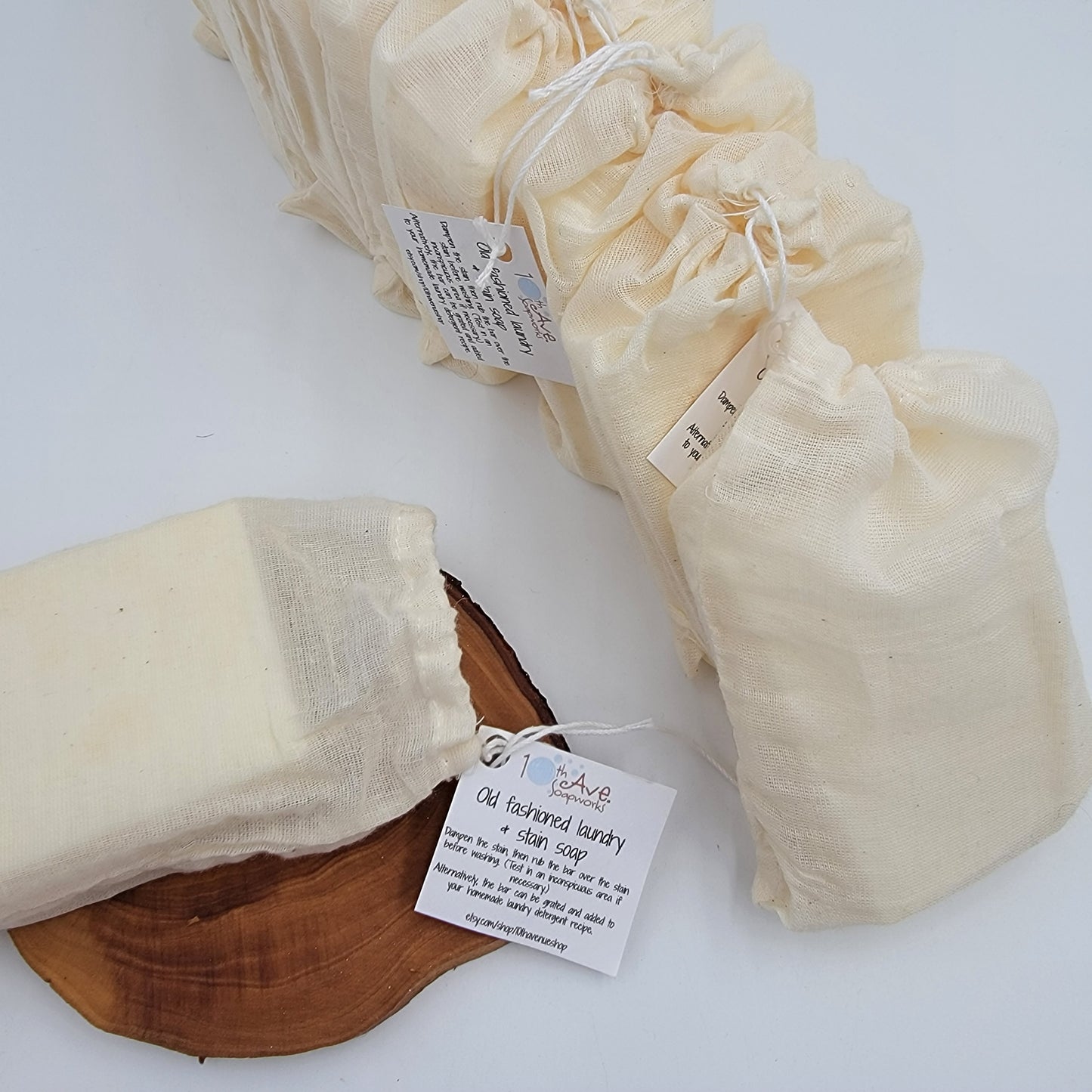The advertisement image showcases an arrangement of six handmade soap bags intended for sale. Each soap bag is composed of white cloth with matching drawstrings and is adorned with a small white tag. The tag reads "10th Ave Soapworks. Old Fashioned Laundry and Stain Soap" in black text, with additional, smaller, unreadable text below. The bags are neatly lined up against each other, resembling a row of standing dominoes, on a white surface, suggesting a table or countertop backdrop. To the left of the image, there's a piece of varnished wood slice, possibly used as a decorative coaster, highlighting one of the soap bags. The varnish darkens the wood but still allows the natural grain to show through, adding an organic touch to the setup. The overall setting is elegantly simple, emphasizing the purity and handcrafted quality of the soap products.